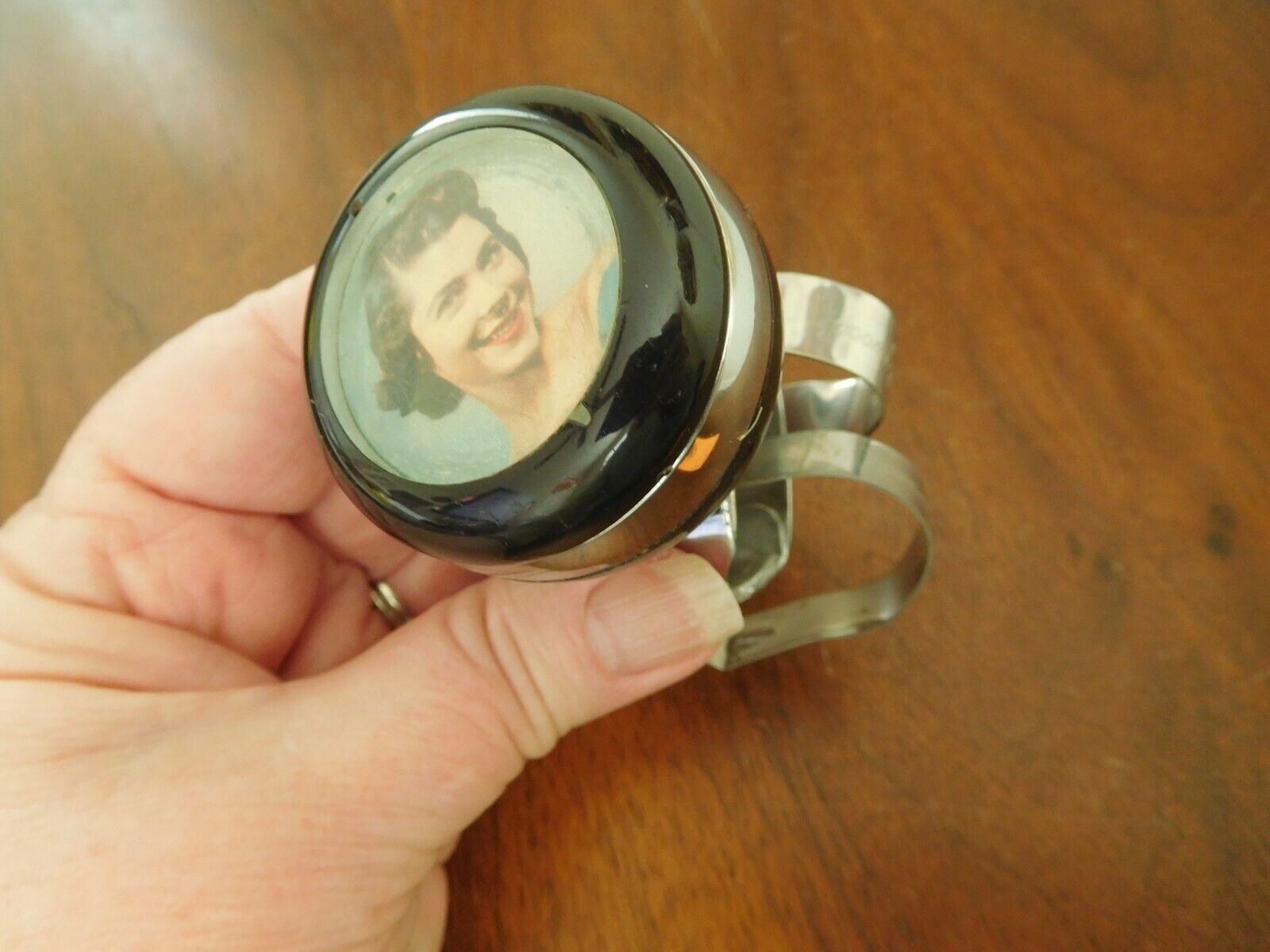This is a close-up photograph of a woman's left hand, adorned with a silver wedding ring on her ring finger. Her hand, with long, manicured nails, lightly tinted or natural, extends from the lower left corner of the image and rests on a medium brown wooden table with visible wood grain. The hand is clutching a round, metallic object that appears to resemble a bicycle bell in size and structure, featuring little curved metal pieces on the back that could clip onto handlebars or clothing. The top of the object has a black rim encircling a vintage portrait of a young woman from the 1940s or 1950s. The woman in the portrait has short, curled hair with bangs, and she is dressed elegantly, exuding an engaging smile with red lipstick, set against a light blue background. The hand and the memento it holds dominate the frame, making the intricate details of both vividly clear.